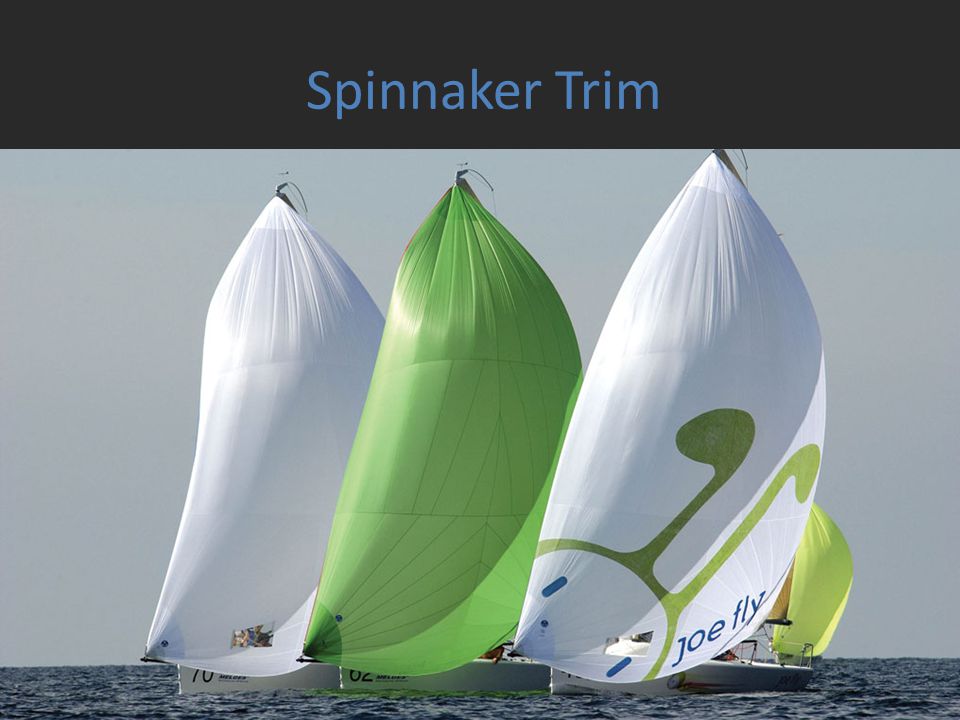The image captures a vibrant seascape featuring three sailboats side-by-side gliding over rippling water under a gray sky. At the bottom of the photograph or video freeze-frame, waves indicate a windy day. The central focus comprises three spinnaker sails unfurled mid-action, with all boats appearing to be of the same model.

From left to right, the sails display distinct colors and designs: the left sail is solid white, the middle sail is lime green, and the right sail is predominantly white with a lime green character featuring two antennae and blue eyes at the bottom, along with the blue text "Joe Fly." There’s also a small light yellow sail visible behind them. 

The horizon cuts across the image about a sixth of the way up, creating a clear separation between the dynamic water and the serene sky. Across the top of the image, a black band features the blue text "Spinnaker Trim."

This visually detailed scene could easily be used in a PowerPoint presentation, showcasing photographic realism and precise typographic design.